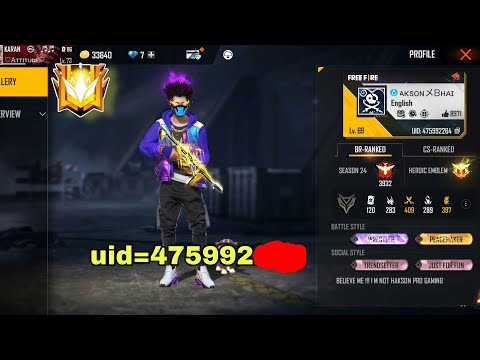The still image, rectangular and wider than it is tall, appears to be a screenshot from a video game, likely "Free Fire." Dominating the center is a drawn character dressed in a blue jacket and black pants, exuding a gangster aesthetic. His black hair is accentuated by purple flames, and he sports a blue face mask. The character wields a golden, futuristic weapon and dons white shoes. 

The left side of the image features a yellow UID number, partially obscured by a red splotch, reading "UID = 475992." Above and to the left of the character is a yellow-gold banner with the partial number "33640" and a heart symbol marked as "7+," suggesting additional hidden information. The background behind the character is dark gray to black, further highlighting his vibrant colors.

On the right side of the image, under the heading "Profile," is detailed game information including "Free Fire," level 69, and rankings for "BR/ranked" and "CS/ranked" in Season 24, accompanied by a heroic emblem. The sidebar also includes various stats, a skull and crossbones, and other emblems. At the very bottom, a text reads, "Believe me, I'm not something pro-gaming." This collection of elements paints a detailed and comprehensive picture of a gaming screen filled with detailed player stats and an emphasis on competitive game rankings.